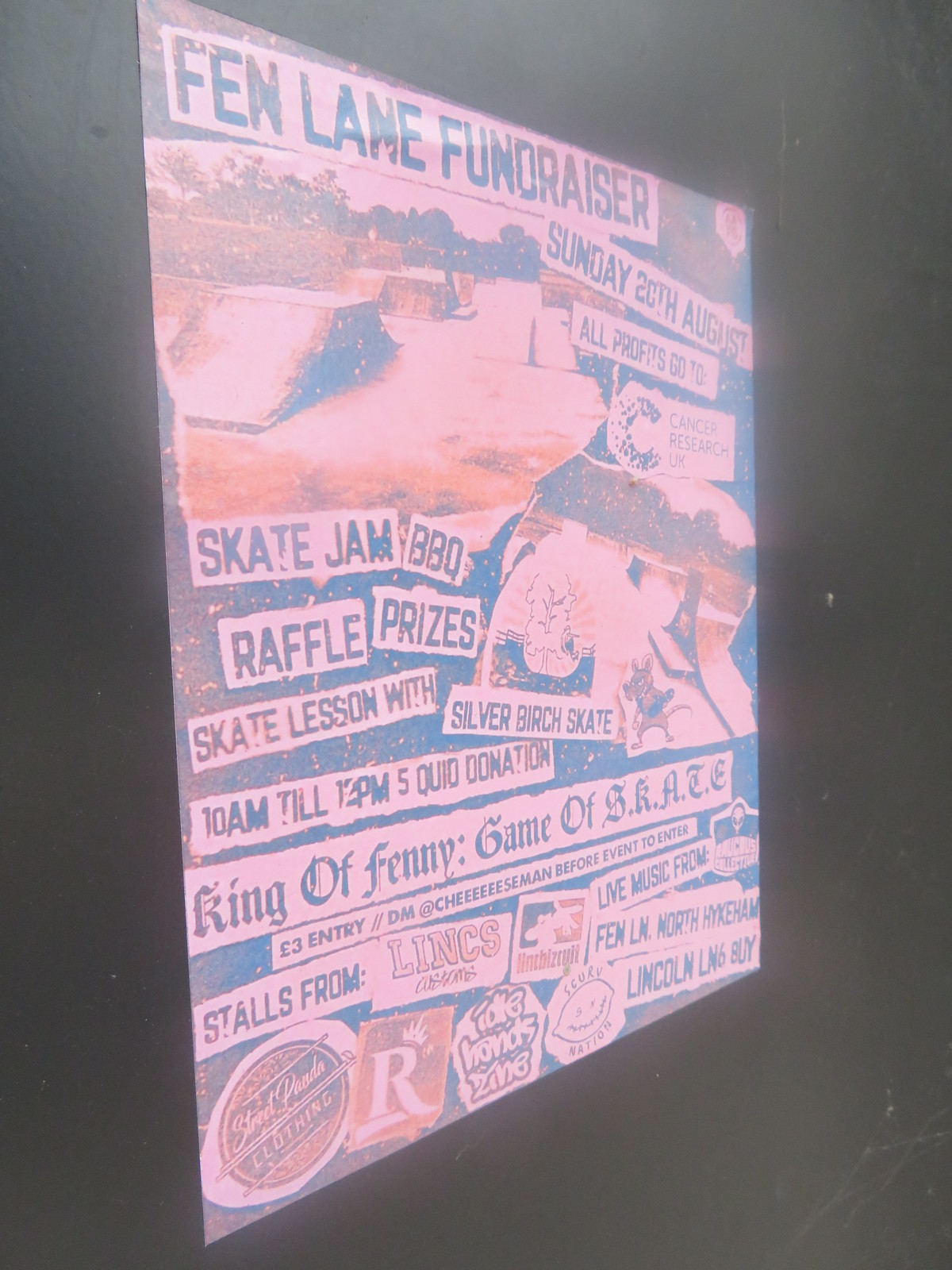The image is a vertically oriented, slightly blurry photograph of an angled poster with a solid black background. The poster is tilted, creating a slant from the left to the right bottom corner, making the bottom run in a rough 130-degree direction. The top of the poster prominently displays the words "Fen Lane Fundraiser," beneath which there is a somewhat washed-out image of a skate park featuring ramps that resemble a flattened pyramid with skateboard ramps on each side and surrounding flat ground. The image has a brownish hue, giving it an old-school look. 

Below the image, the poster announces, "Sunday 20th August," followed by the text, "All profits go to Cancer Research UK." On the left side below this, the poster details various event activities: "Skate Jam, Raffle, BBQ Prizes, Skate Lesson with Silver Birch Skate," with the timing mentioned as "10 a.m. till 12 p.m.," and a donation fee indicated as "5 quid donation."

Further down, the text reads "King of Fenny game of SKATE," along with an entry fee. The bottom of the poster features sponsor logos, including Lynx and a capital 'R'.

Overall, the poster is promoting a charity skateboarding event with various activities and sponsor logos, despite its somewhat blurry and washed-out appearance.